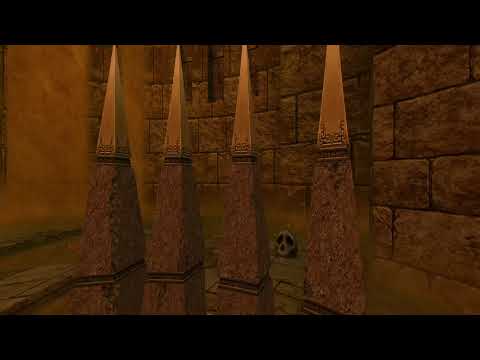The image is a surreal, possibly animated or digitally rendered scene, set outside in front of a building at night with very little lighting. The photo features a black border on the top and bottom, and the central focus is on four tapered, stone buttresses or pyramidal pillars that rise towards the top of the image. The stone material is predominantly gray with golden or brownish-orange light illuminating the upper sections of the pillars, giving them a fantasy-like appearance. The scene is reminiscent of an ancient or historical site, such as an Egyptian temple, possibly indicating a digital fantasy environment. The space appears cavernous, akin to a cellar or temple interior, with large, rusticated stone walls surrounding the pillars and forming the structure's perimeter. There are no people or text present in the image. Between two of the pillars, a skull is notably visible, adding to the eerie and mysterious atmosphere of the scene.